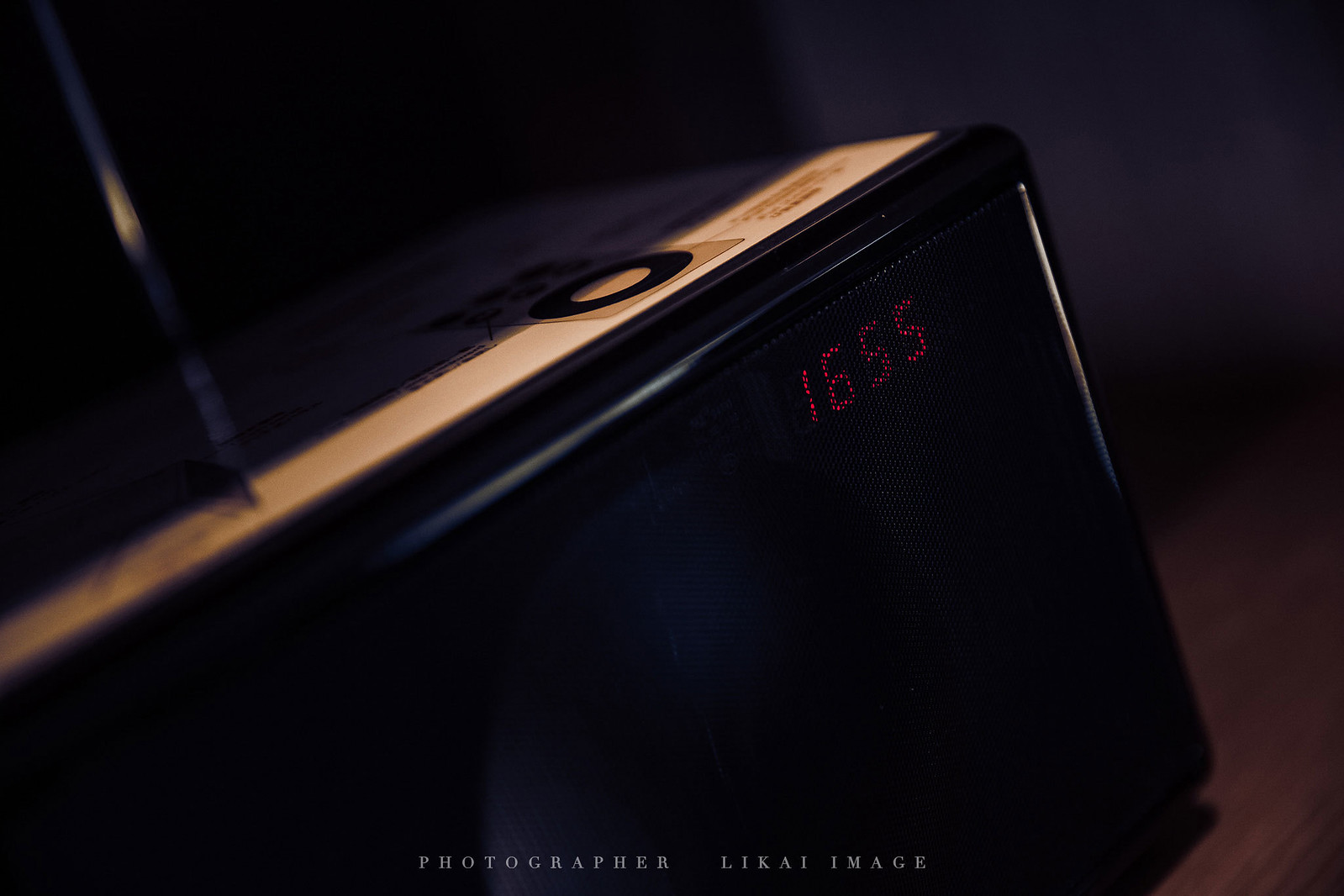The artistic photograph, attributed to photographer Lakai image, captures a dark, moody scene of a classic electronic device with a sophisticated design. Positioned on a lightly colored wooden table, the device features a light wood casing that adds a touch of elegance. A notable detail is the red digital display on the front, showing the time "1655," partially obscured by a black grating. A silver top with various buttons and an antenna protruding from it is visible, casting a shadow over the device. The background is intentionally blurred to create a dramatic effect, enhancing the focus on the electronic equipment. The overall composition emphasizes the juxtaposition of modern technology with vintage aesthetics.